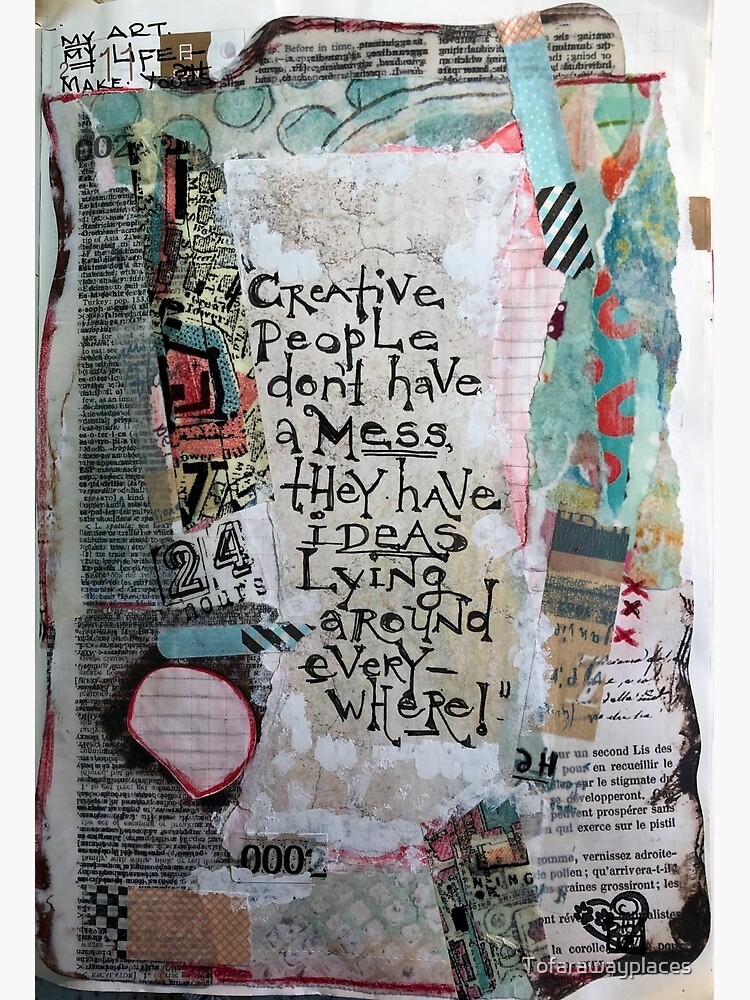The image is a vibrant collage of magazine, newspaper cutouts, and book pages layered intricately on top of each other. At its heart, a piece of light beige paper features a prominent quote in black text: "Creative people don't have a mess; they have ideas lying around everywhere!" This serves as the central theme of the artwork. Surrounding this message are varied elements including blue circles, black stripes on blue backgrounds, and red circles on blue backgrounds, contributing to the rich tapestry of the piece. In the top left-hand corner, handwritten in black pen, it says, "My Art, My Life." Additional elements include a "24 hours" label, a "0002" sticker, and a piece with orange diagonal lines. The bottom right-hand corner houses text saying, “Too far away places,” alongside fragments of text in another language. The overall aesthetic is a testament to the creative chaos, with book pages marked by white backgrounds and black text, blending seamlessly with various other visual elements.